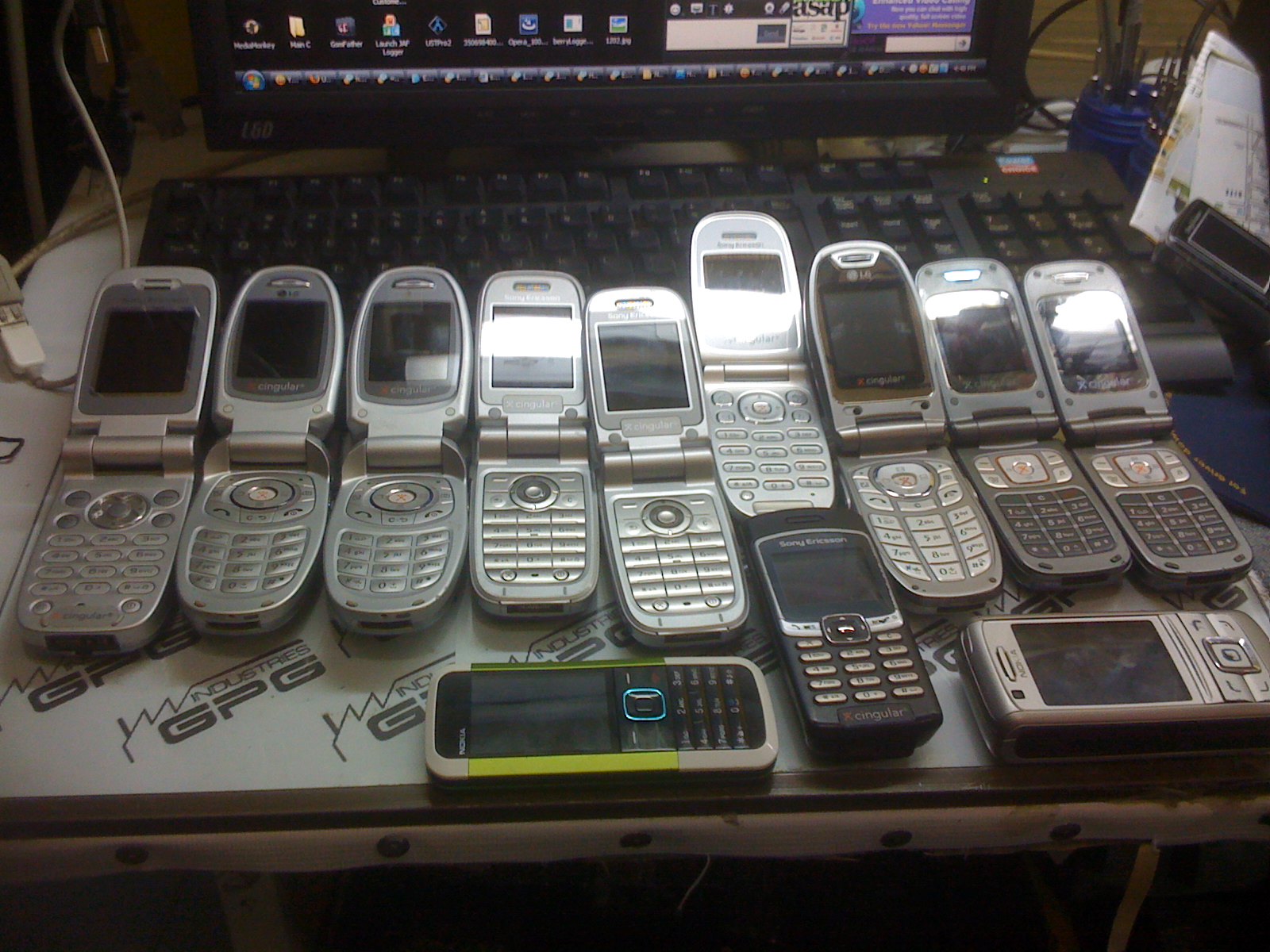The photograph showcases a nostalgic collection of a dozen old-style cellular phones from the 90s and early 2000s, meticulously arranged on a desk. Nine of the phones, varied in design with some more square and others more oblong, are classic flip phones, all flipped open and slightly staggered in their alignment. In front of these, on the right side of the desk, sit three non-flip phones, notable for their thick, blocky build and square screens, reminiscent of early BlackBerry devices. Behind this array of vintage phones, a black computer keyboard is visible with the upper halves of the flip phones' screens resting on it. The scene is set against the backdrop of a computer monitor, which is on, displaying a dark taskbar filled with indistinct icons and larger icons scattered across the screen. The surface of the desk beneath this display is white and features a black graphic that reads "Industries GPG." The overall scene is a sentimental nod to old mobile technology, capturing the essence of early cellular innovation.